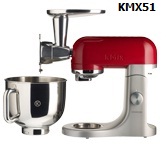This image displays a detailed view of a kitchen mixer set against a white background. Positioned in the upper right corner, black text reads "KMX 5-1." The main focus on the left side of the image features a large, shiny metal mixing bowl equipped with a sturdy handle, designed to connect seamlessly to the mixer. The mixer itself, located to the right of the bowl, has a distinctive red top that is rectangular with rounded edges. A silver piece extends downward from the red top, creating a connecting platform that appears almost cylindrical, culminating in a uniquely designed boot-shaped housing with a circular cut-out at the base. This silver-lined cut-out allows the bowl to attach securely. Midway up the red section is a round switch, adding functionality to its sleek design. The mixer, elegant in its stainless steel build, combines both aesthetic appeal and practical use.